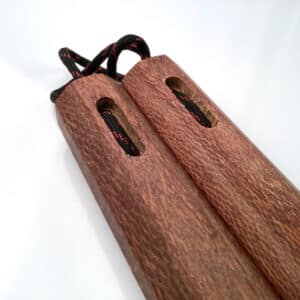The image depicts a close-up view of a handcrafted set of wooden nunchaku, positioned diagonally from the bottom right to the top left at a 45-degree angle against a predominantly white background. The photograph itself is quite small and square. Both wooden handles of the nunchaku are cylindrical and closely aligned. Each handle features a very narrow, tall, oval-shaped hollow indent near the top, within which a black and red nylon rope is visible, connecting the two sections. The handles exhibit fine details and a grip texture that could suggest they are aged and might have been used for physical activities like martial arts or exercise, possibly in an educational setting. The overall image is clear, brightly lit, and free of any text, numbers, or people.